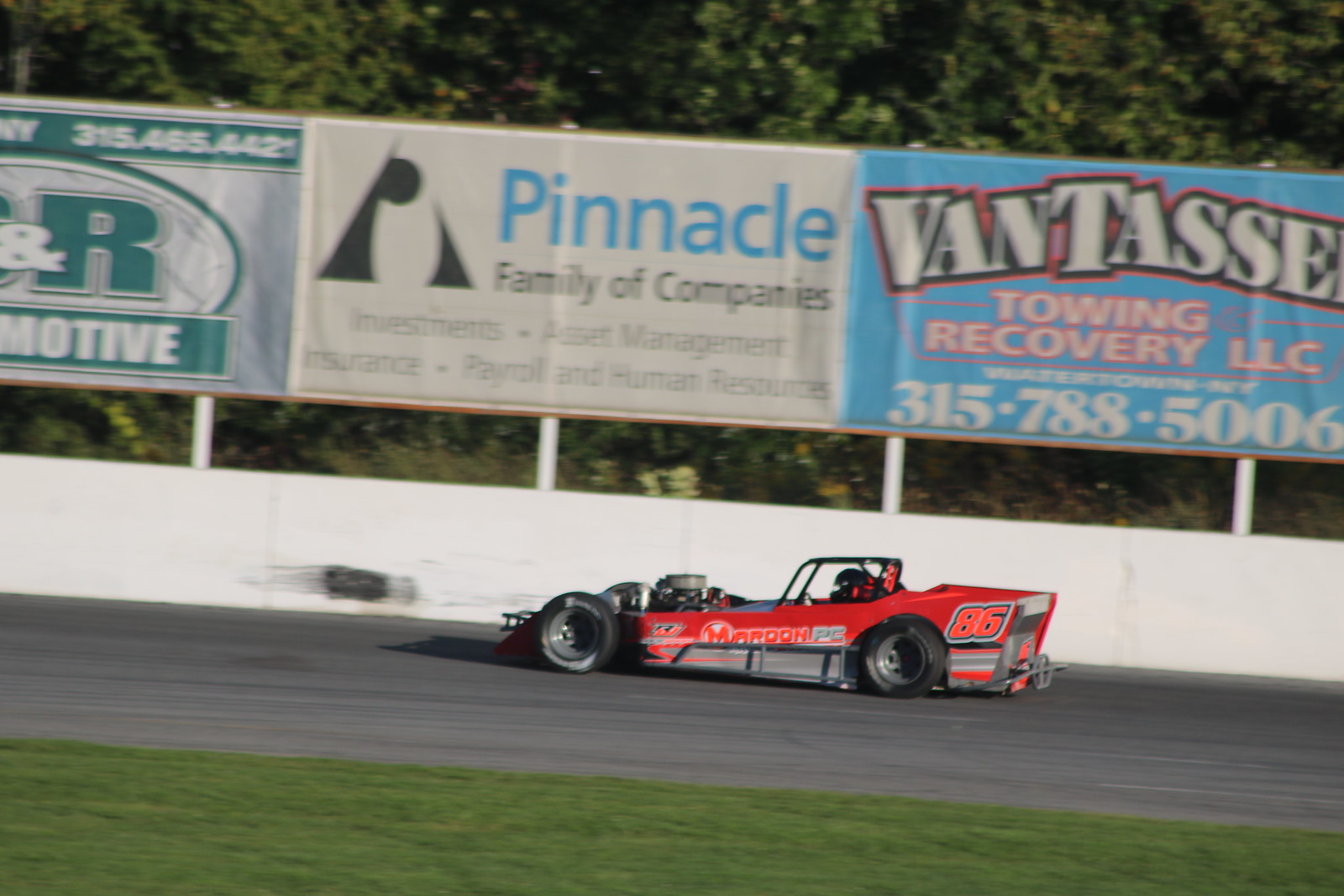The image depicts an outdoor scene set at a racetrack, featuring a vivid depiction of a racing event. Dominating the scene is a sleek, red Formula One-style race car, marked with the number 86 in red on the back. Details on the car reveal a sponsor logo reading "Maproon PC-86," with a glimpse of the driver wearing a black helmet visible inside the low-to-the-ground, open-topped vehicle.

In the foreground, a strip of green grass lines the bottom of the image, transitioning into the dark asphalt of the racetrack. The car races along this track, framed by a white barrier positioned behind it. Rising above the barrier are several billboard signs: one prominently displays "Pinnacle Family of Companies," another reads "Van Tass Towing Recovery LLC 315-788-5006," and additional ads highlight investments, asset management, insurance, payroll, and human resources.

The background of the image is rich with greenery, showcasing an expanse of green trees and bushes under a clear sky. The primary colors in the scene include vivid red from the car, various shades of green from the grass and trees, stark white from the barrier, and the textual pops of blue and other colors on the car and advertisements. Overall, the image captures the high-speed drama and commercial vibrancy of a racetrack environment on a clear day.